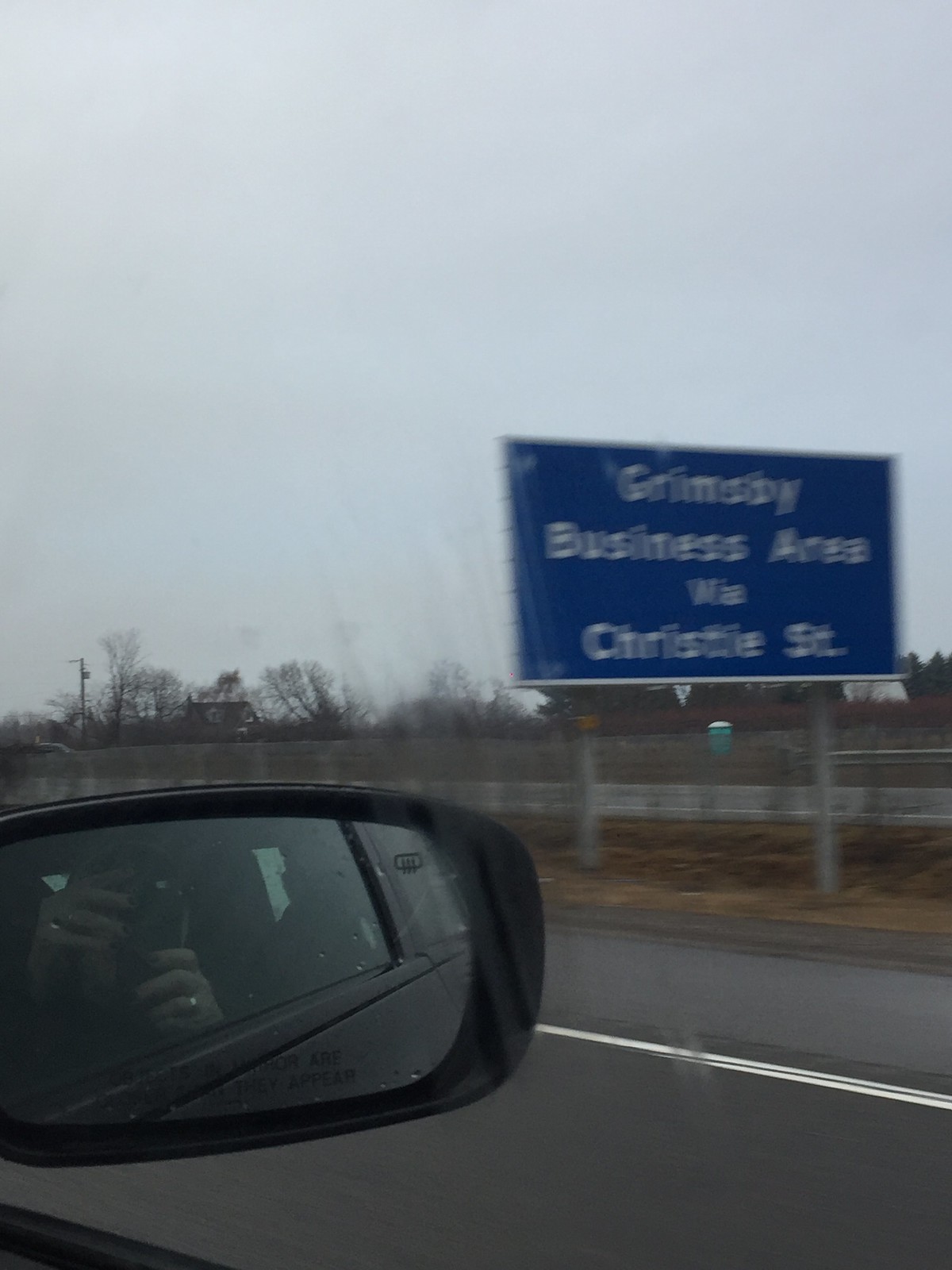The image, taken from the passenger side window of a car, captures the rearview side mirror in the left-hand corner where a person is seen holding up their phone, taking a picture of the scene. The reflection suggests the person is inside a black car. The view through the window shows an out-of-focus blue street sign that possibly reads "Grimsby Business Area" and "Christie St." Beyond the sign, the blurred exterior reveals a brown field bordered by some trees and a small house in the distance. The upper half of the picture is dominated by a dull, gray sky, lending a muted tone to the overall scene.